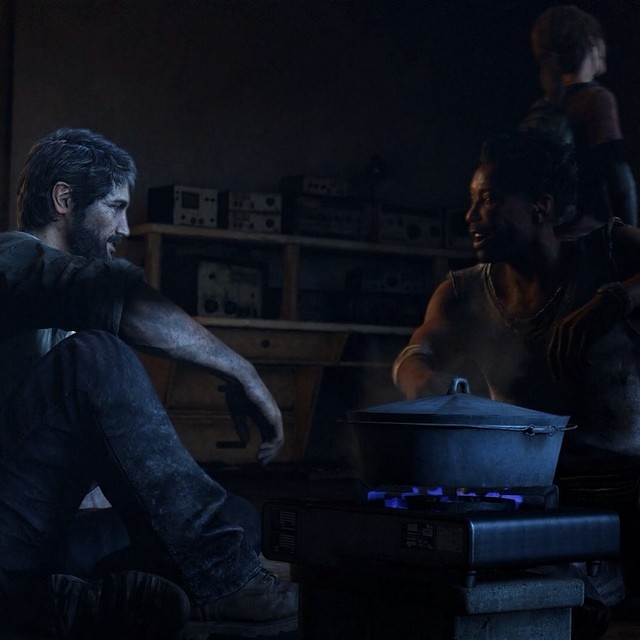In this still shot from a video game, a man with short black hair and a black beard is seated on the floor, his right arm resting on his right knee. He is dressed in dirty jeans and brown boots. To his right, another man in a gray tank top, with a bandage on his arm, tends to a gray pot heating on a stove with blue flames flickering beneath it. The background features a brown shelf filled with various boxes. Behind the seated man, another person is standing, wearing a backpack and a red T-shirt layered over a white long-sleeve shirt. This individual, with dark brown hair pulled back into a ponytail, appears to be gazing at the wall or possibly looking outside.